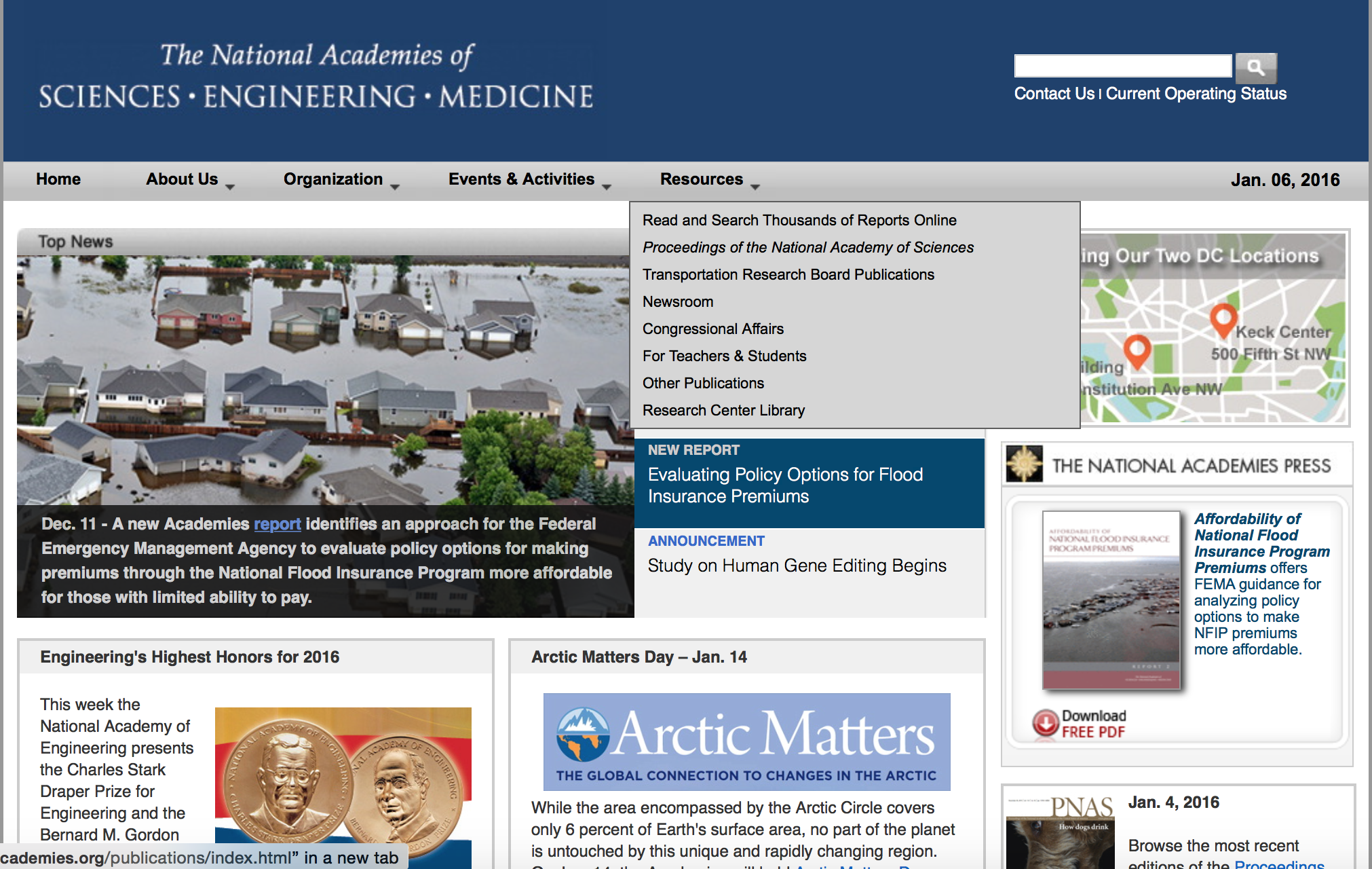This photograph captures a webpage from the National Academies of Sciences, Engineering, and Medicine. In the upper left corner, the organization’s emblem is clearly visible. The image features a blue navigation bar spanning the width of the page with a search bar positioned on the right side. Directly below this, there is a gray menu bar with various tabs: Home, About Us, Organization, Events and Activities, and Resources. To the far right of the gray bar, the date "January 6, 2016" is displayed. The Resources tab includes a dropdown menu with multiple options: "Read and Search Thousands of Reports Online," "Proceedings of the National Academy of Sciences," "Transportation Research Board Publications," "Newsroom," "Congressional Affairs," "For Teachers and Students," "Other Publications," and "Research Center Library." The website also features a section under the top bar for "Contact Us" and "Current Opening Status."